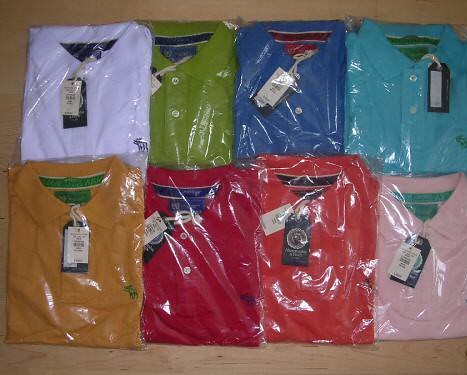The image displays a meticulously arranged collection of eight collared shirts, each neatly folded and carefully wrapped in clear plastic film with white and black tags attached, indicating uniformity and potential brand consistency. These shirts are laid out on a light oak-finished wooden table adorned with darker semi-circular patterns. The shirts, likely intended for a product listing, are organized in two rows of four. The top row, from left to right, features shirts in light purple, green, blue, and light blue. The bottom row includes shirts in dark orange, red, another dark orange, and pink. Each shirt sports a collar and a few buttons, characteristic of polo shirts, and some have subtle logos, including one depicting a moose on the orange shirt.